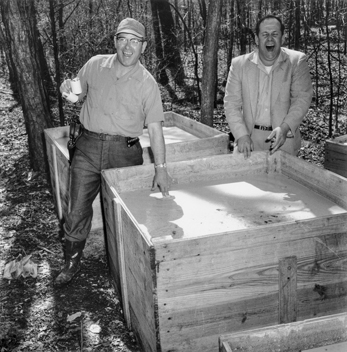In this black-and-white vintage photograph, two Caucasian men are standing outdoors in a forest area, surrounded by tall trees and a ground covered with mulch, dirt, and leaves. The men are positioned in front of three large, square, wooden crates, with two crates prominently visible and the third one barely discernible in the background. The man on the left is dressed in a light short-sleeved, collared shirt, dark trousers, and boots, complemented by glasses and a hat. He has a broad smile and one hand placed on one of the crates. The man on the right, adorned in a light-colored suit, white button-down shirt, dark belt, and light trousers, stands with his eyes closed and mouth open in laughter. Their evident joy and camaraderie are captured against the rustic, serene backdrop of the forest.